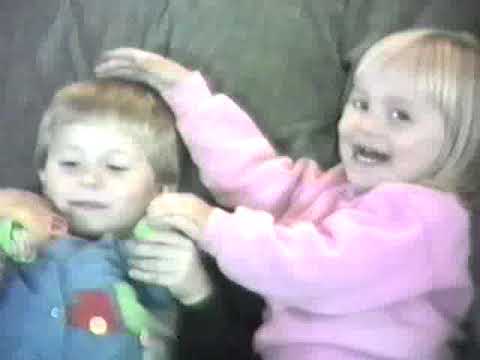This is a small, square, grainy photograph featuring two young children. The child on the right is a little girl with short blonde hair, wearing a long-sleeved, light bubblegum pink sweater. She is smiling broadly at the camera, revealing her teeth, and her dark eyes twinkle with joy. The left side of her body is facing the camera as she leans towards the smaller boy on her left. Her right hand is gently patting the boy's head, and her left hand appears to be holding or hovering around the same area. The boy, also blonde, looks slightly younger and is wearing a blue shirt with a truck design on the front. Although he is not smiling, he looks content as he looks down at an object he holds in his left hand, which appears green. The children are lying back on what seems to be an olive-green blanket or couch, providing a cozy and intimate backdrop to this candid and cheerful moment.